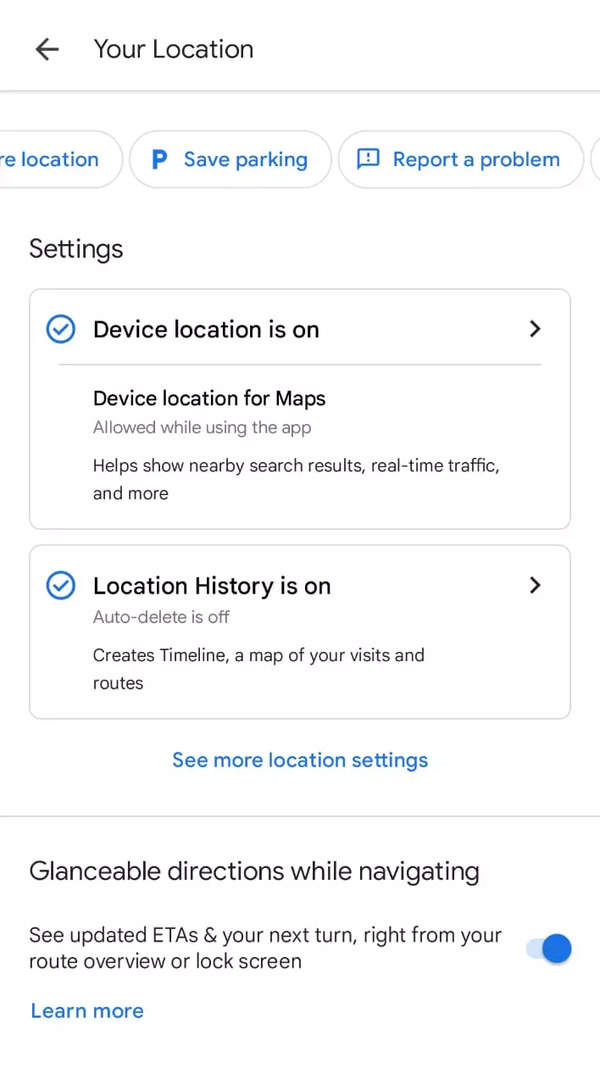This image displays a smartphone screen showcasing a location settings page. The top section features a left-facing arrow beside the text "Your Location," both in black on a white background. Throughout the entire image, the background remains white, providing a clean and consistent look.

Below the header, there is a horizontal scroll bar consisting of elongated circles featuring blueprint-style icons and options like "Safe," "Parking," and "Report a Problem." Two additional circles are partially visible, one with its text cut off and the other showing just the edge of the circle.

Further down are two settings boxes. The first box indicates that "Device location is on," marked with a checkmark inside a circle. To the right is a partial right-facing arrow along a thin line. Beneath this, it reads "Device location for maps."

The second box operates similarly, stating "Location history is on," also accompanied by a checkmark inside a circle and the partial right-facing arrow. Below these boxes, in blue text, it says "See more location settings."

Following this section, a thin gray line separates it from the next part, which reads "Glanceable directions while navigating: See updated ETAs and your next turn right from your route overview or lock screen." An on-off slider is located to the right, shown in the "on" position with a bright blue circle confirming its active status.